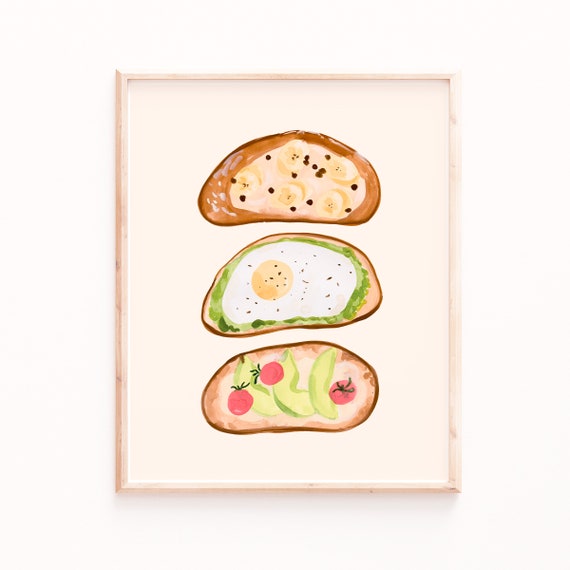Framed within a thin, light wood-colored, beveled frame, this vertically oriented kitchen wall art depicts an abstract trio of toast illustrations. Set against an off-white to subtly pinkish-beige background that gradates lighter towards the bottom, each of the three vertically-stacked toasts is meticulously detailed. The top slice features a slice of brown bread slathered with peanut butter, topped with banana slices, and scattered with small chocolate dots. The middle toast showcases a sunny-side-up egg with a vivid yellow yolk, set on a bed of guacamole and sprinkled with black pepper. The bottom toast is adorned with avocado slices and halved cherry tomatoes. This artistic arrangement is held against an eggshell white background, creating a homely yet elegant piece perfect for a kitchen setting, mounted on an off-white wall.